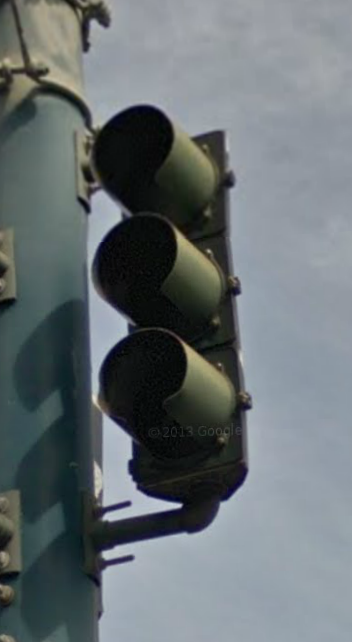This close-up digital photograph captures a traffic light mounted on the side of a green metal pole, rather than suspended from overhead wires. The pole, which extends above the traffic light, has additional metal pieces and piping attached to it. The traffic light itself is painted a dark, grass-colored green, matching the pole it's attached to. None of the traffic lights—red, yellow, or green—are illuminated in the photo, likely due to the angle of the shot. The copyright notice, "2013 Google," is faintly visible in light white font towards the bottom of the image. The background features a partly cloudy sky with a mix of gray and pale blue, further diffusing the traffic light's visibility. Shadows cast by the sun add depth to the scene, highlighting the structure's metallic components.